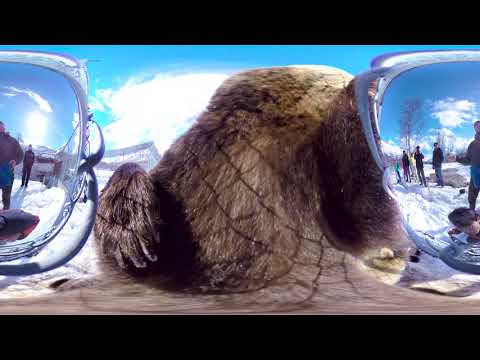In this highly edited, vertical rectangular image, black stripes run horizontally across both the top and bottom. The scene is divided into three main sections. On the left and right sides, there are mirrored images that appear to be encased in a clear, curved plastic resembling the material of sunglasses lenses. These sections show groups of people standing in snowy terrain, all dressed in winter clothing with jackets and pants. The sky behind them is a vibrant blue with scattered clouds, and some bare trees can be seen in the background.

In the center of the image is a large, brown, furry animal with a dark brown tail. Only one of its clawed paws is visible, showing three long nails, but its head and neck are obscured, making identification difficult. The central figure is placed against the same blue sky background as the side images. Altogether, the entire composition rests on a brown platform, creating a surreal, staged appearance as if capturing a scene outdoors in winter, possibly near someone's home. The setting is bright and daytime, emphasizing the snowy and cold environment.